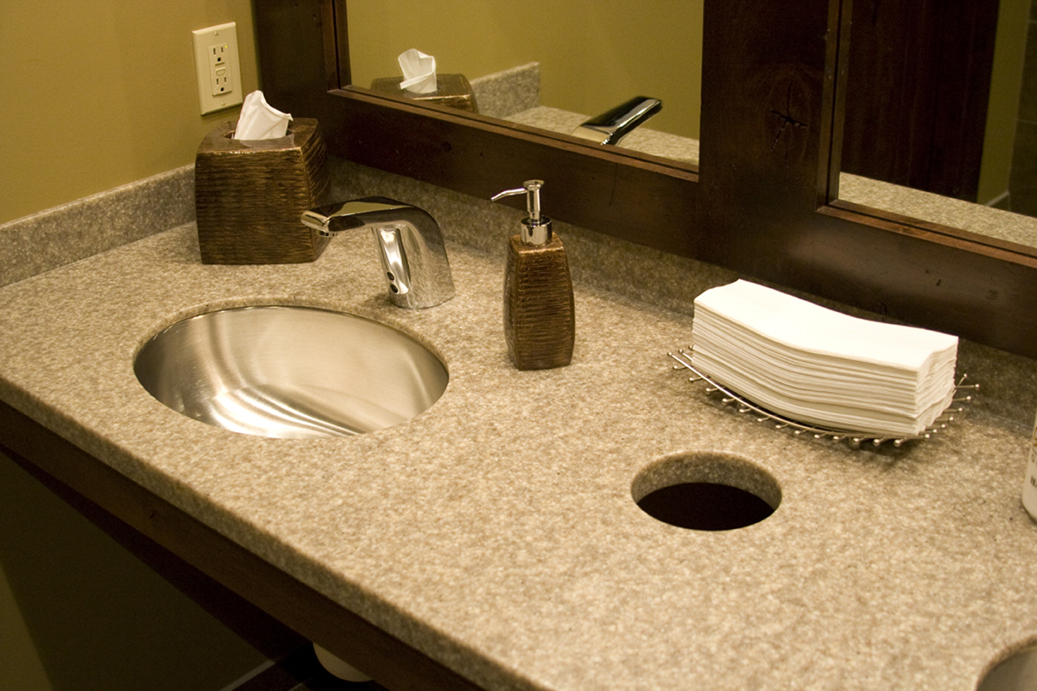This photograph captures an indoor bathroom vanity, characterized by a modern and functional design. The focal point is a gray countertop adorned with white and brown speckles, adding a touch of elegance to the space. Positioned in the left corner of the counter is a box of tissues encased in a stylish brown tissue cover. Just above the counter, an electrical outlet is conveniently placed next to the mirror, which features a charming wood frame and is notably split into two sections.

The vanity includes two sinks, with the right-hand sink visible at the bottom-right corner of the image. This sink's basin is clearly shown in the frame, and there is a hole drilled into the center of the countertop, likely intended for plumbing connections or additional fixtures. Behind this hole, a neat stack of paper towels rests on a metal wire holder, ensuring easy access for users.

Further enhancing the vanity's functionality is a container of soap positioned to the right of the visible sink. The sink itself is equipped with a sleek silver spigot head, designed without knobs to indicate its motion-activated mechanism, providing a touchless and hygienic hand-washing experience. This carefully arranged setup combines practicality with aesthetic appeal, making it both a utilitarian and visually pleasing bathroom space.